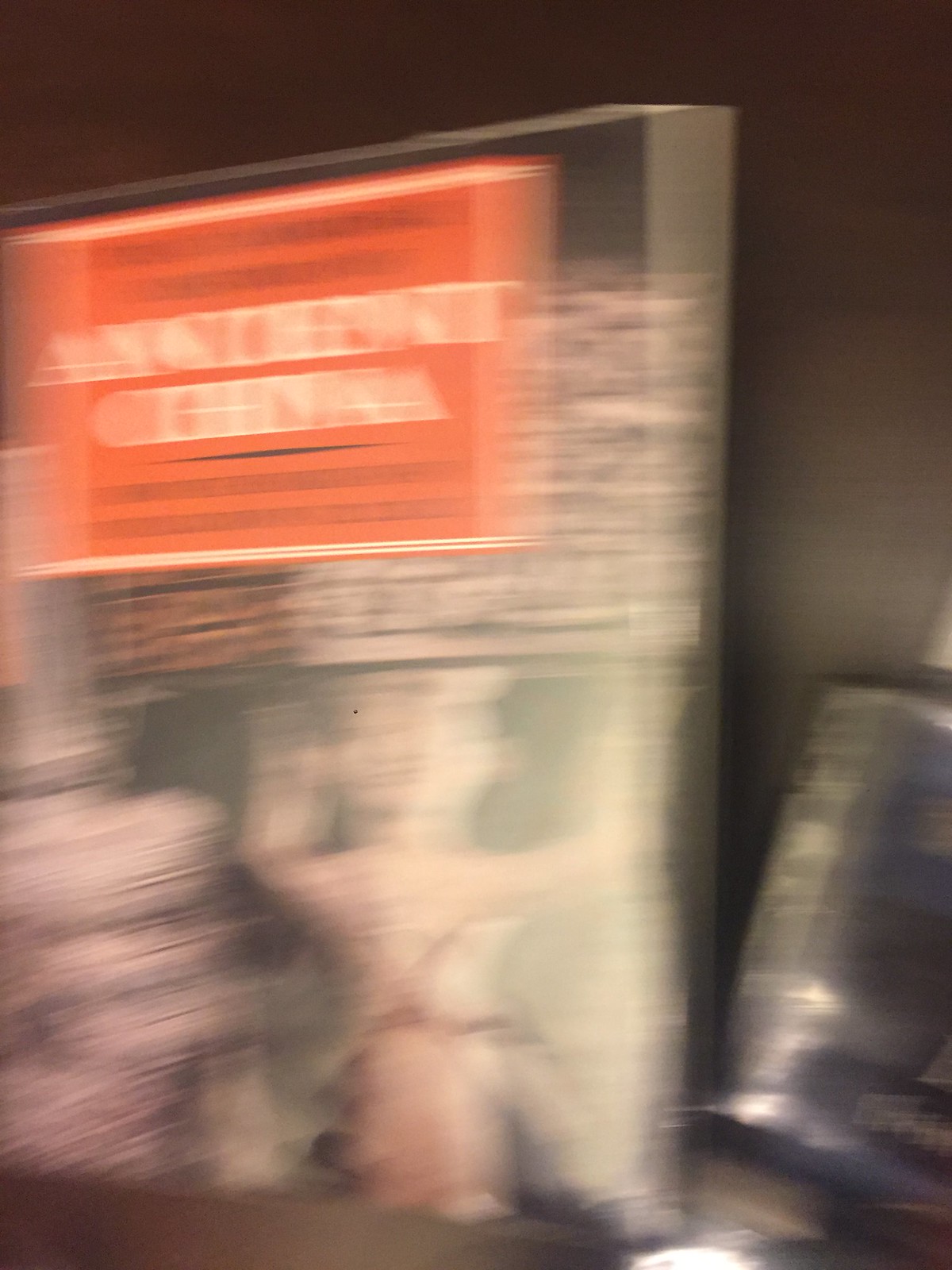The image is a very blurry color photograph featuring what appears to be a book or DVD with a prominently displayed title that reads "Ancient China." This title is situated within an orange rectangle at the top of the image, outlined in white, with some additional black text appearing above and possibly below the main title. Due to the blurriness, the background details are indiscernible, but there seems to be an illustration of a person or figurine with raised hands, hinting at a theme related to ancient artifacts or archaeology. The overall background is dark gray, accompanied by streaks of light and a mix of colors, including pastel green, red, and purple hues.

To the right of the central item, there is an oblong, slightly rounded object that might be a vessel or a metal container, resembling a pewter bowl or possibly a pair of binoculars. This object appears to be predominantly blue with some gold or brass-colored detailing, and there's also something gleaming white or silver at the bottom of the image. Despite the heavy blurring, the mixture of traditional elements and colors likely aims to evoke a sense of ancient China and its treasures.